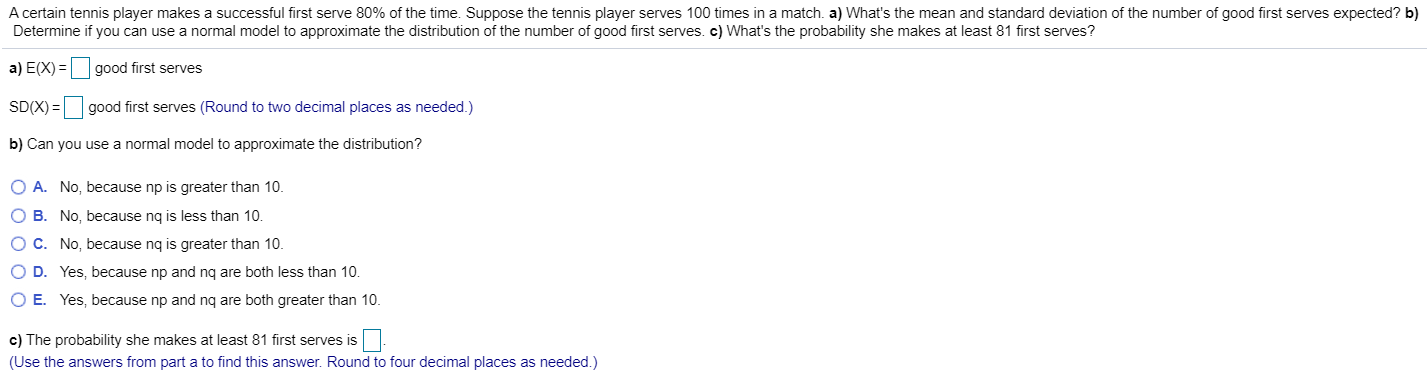**Detailed Caption:**

This image is a screenshot of an academic quiz application focused on a mathematics problem pertaining to probability and statistics. The problem is displayed in black text on a clean white background. It involves a scenario where a tennis player successfully makes a first serve 80% of the time. The problem is broken down into three main parts:

1. **Part A** asks for the mean and standard deviation of the number of successful first serves out of 100 attempts in a match. The text prompts the user to enter these values in a format: "mean = ___ good first serves" and "SD = ___ good first serves," with instructions to round the answers to two decimal places.

2. **Part B** requests an assessment on the applicability of a normal model to approximate the distribution of successful first serves. It provides multiple-choice options:
   - A) No, because NP is greater than 10.
   - B) No, because NP is less than 10.
   - C) No, because NQ is greater than 10.
   - D) Yes, because NP and NQ are both less than 10.
   - E) Yes, because NP and NQ are both greater than 10.

3. **Part C** inquires about the probability of the tennis player making at least one successful first serve, phrased as: "The probability she makes at least 01 first serves is ___."

The structured problem presentation indicates a thorough assessment of statistical knowledge, particularly in mean, standard deviation, and the application of the normal model in probability distributions.